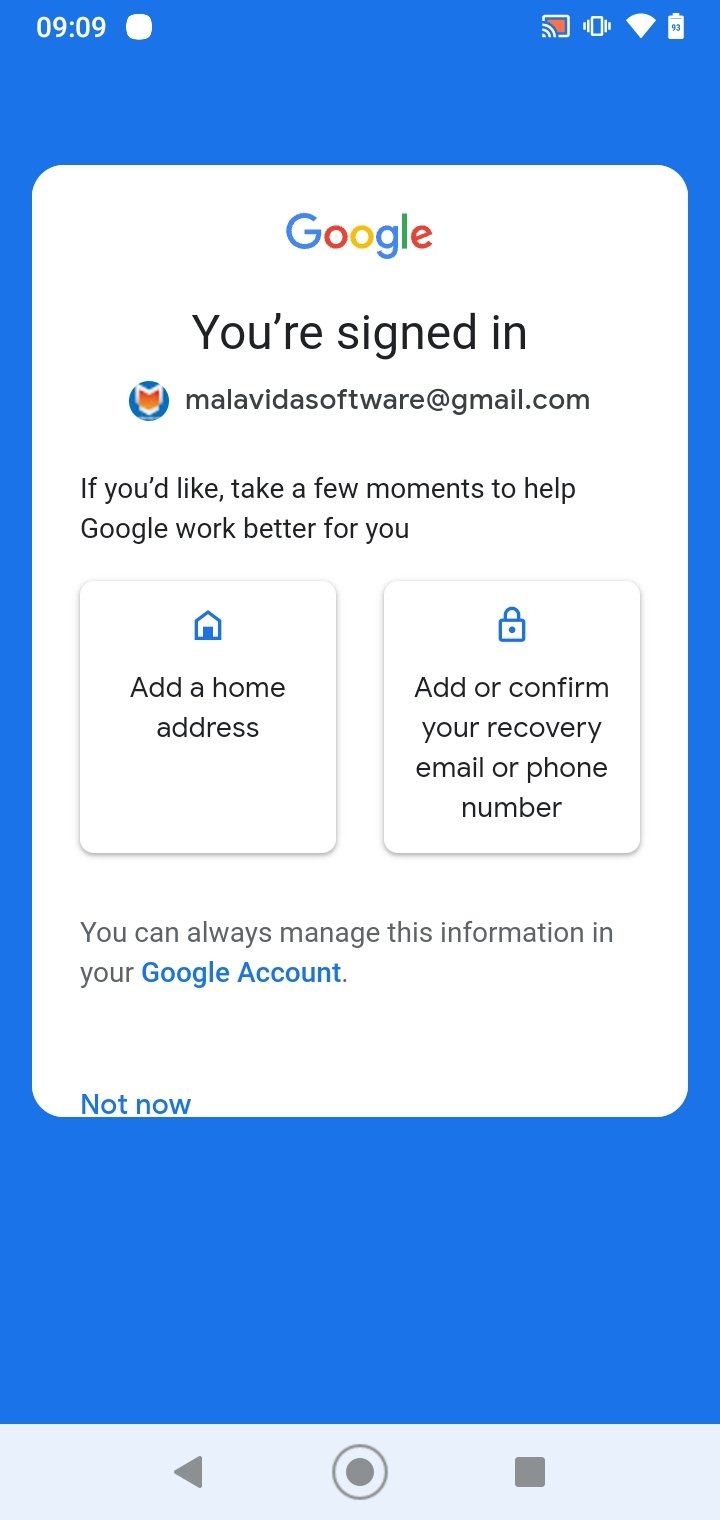This vertical rectangular image features a bright blue background. At the top left corner, there is a time display reading "09:09" with a filled white circle to its right. Along the top edge, a series of small icons is present, the last of which is a battery icon depicted in white.

Slightly above the center, closer to the top edge, there is a white rectangular area with rounded corners. At the top of this area, the word "Google" is displayed in its distinct multi-colored letters. Below this, in larger black font, the text reads "You're signed in." Beneath this text, aligned to the left, is a small emoji or icon. Next to this, in black font, is an email address: "malavidasoftware@gmail.com".

Following the email address, there is a message in black font: "If you'd like, take a few moments to help Google work better for you." Below this message are two smaller vertical rectangular areas placed side by side. The first box features a turquoise house icon with the text "Add a home address" in black font underneath it. The second box displays a turquoise security lock icon with the text "Add or confirm your recovery email or phone number" in black font beneath it.

Further down, there is a note in black font that says, "You can always manage this information in your," followed by "Google Account" in turquoise. At the very bottom of the white area, the option "Not now" is written in turquoise.

At the absolute bottom of the image, in an off-white section, there are navigation icons: a left arrow, a circle around a dot, and a filled square.